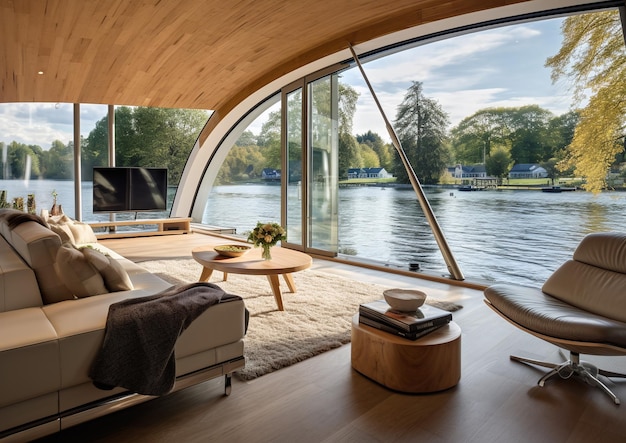The full-color photograph, taken indoors with natural light, is clearly a professional and staged shot of a luxurious living room aboard a high-end yacht, evidenced by the immediate proximity of water visible right outside the large, expansive window. The window extends from the upper right corner to the left of the center, offering a panoramic view of a serene body of water, shoreline, multiple dark trees, and a tree with yellow leaves in the upper right corner. Across the water, several white houses are nestled along the shoreline, framed by a backdrop of trees.

Inside the living room, the interior showcases elegant furniture on a polished wooden floor. A light brown sectional sofa is positioned on the left, facing a center coffee table resting on a white throw rug. There is a large flat-screen TV to the left side, slightly oriented toward the sofa, with an entertainment center beneath it. On the right-hand side of the room, a leather swivel chair sits adjacent to a small table featuring neatly placed books. This sophisticated setting suggests a luxurious lifestyle, further underscored by the pristine and well-appointed decor of the living space.